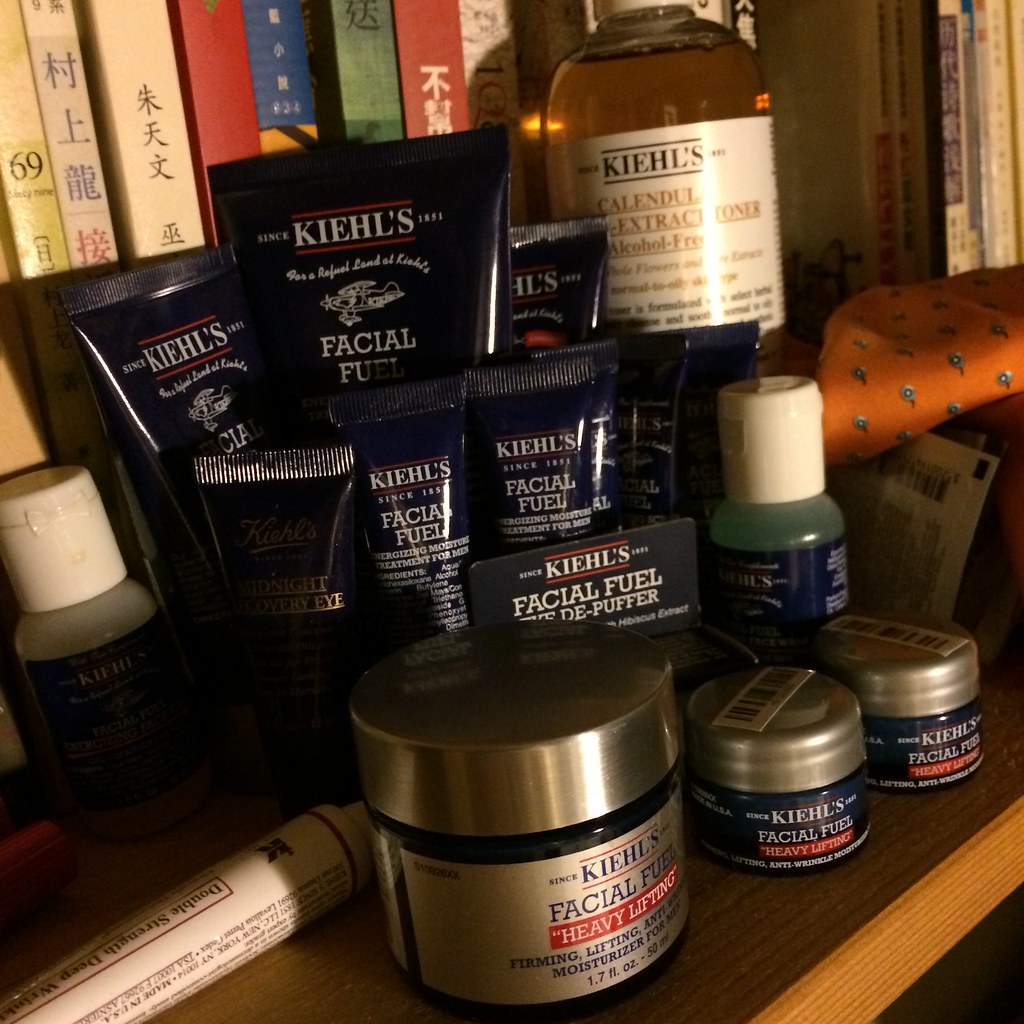The square color photograph captures a meticulously arranged display on a wooden table, presenting an assortment of skincare products. Dominating the scene are various items from the "Facial Fuel" line by Kiehl's. The arrangement is centered around several plastic bottles with serrated tops and text labels. Positioned prominently at the front are three cylindrical glass bottles, with the larger bottle flanked by two smaller ones.

To the left and right of the composition, lotion and liquid bottles enhance the sense of abundance. A notable feature is the large glass bottle labeled "Kiehl's" at the top. Specific product descriptions such as "De-Puffer" and "Heavy Lifting" are visible on some bottles, adding to the context.

In the bottom left corner, a long tube lies diagonally, contributing to the dynamic layout. Behind the skincare products, a bookshelf with colorful book spines and some Asian text serves as an intriguing backdrop. An orange handkerchief draped gracefully at the top right side of the image introduces a splash of color and texture, positioned slightly above the center line.

The entire setup is bathed in overhead lighting, casting soft highlights that accentuate the labels and shapes of the bottles, enhancing the inviting appeal of the still life arrangement.